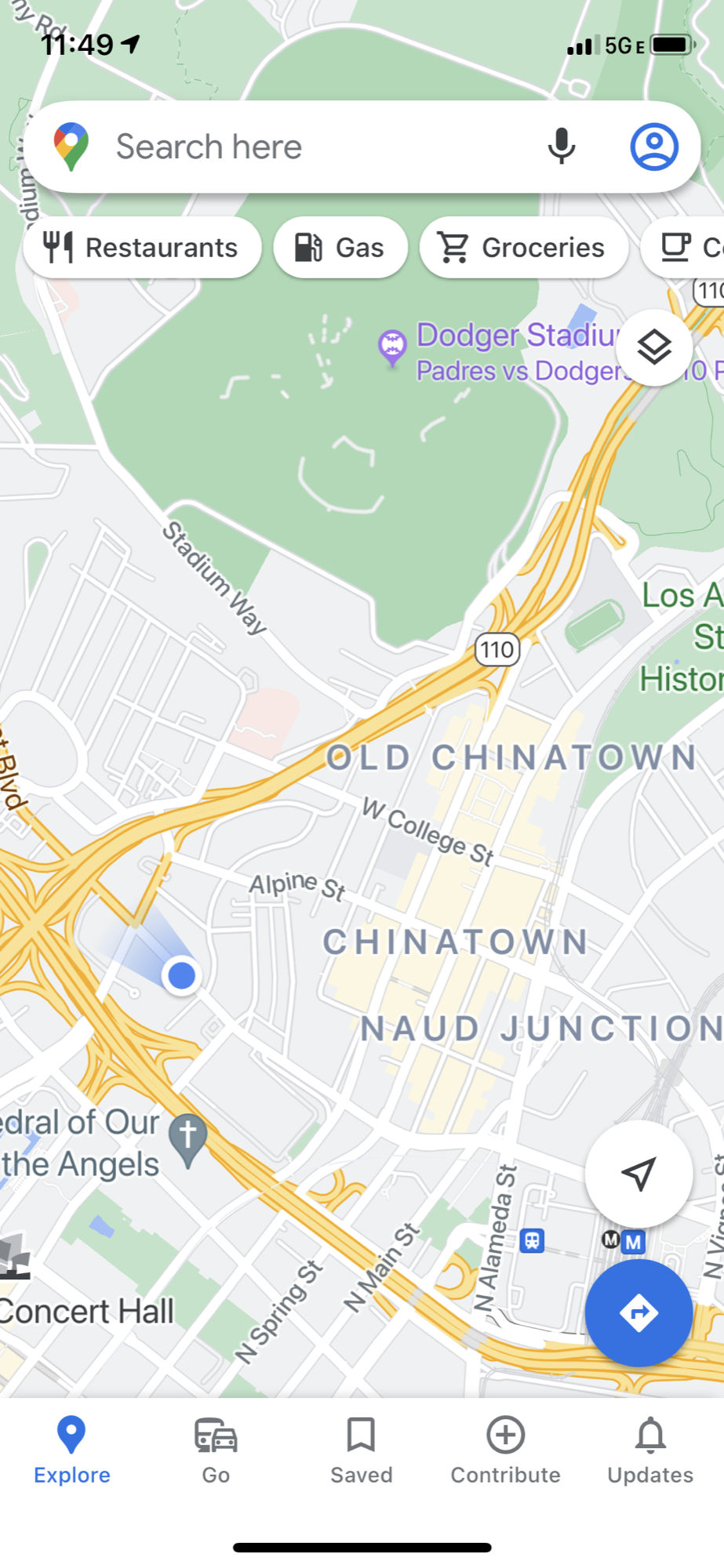The image shows a screenshot of Google Maps on a smartphone. In the upper left-hand corner of the phone display, there is an indicator showing the time as 11:49 AM in black text. A diagonal arrow points towards the right side of the screen. Next to the time, the phone's status bar indicates three out of four bars for signal strength, labeled as 5G, with an 'E' symbol and a black battery icon indicating charge status.

At the top of the Google Maps interface, there is a white oval containing a search bar that reads "Search here" in gray text, accompanied by a gray microphone icon for voice search. To the right of the search bar, there is an outline of a blue circle. Below this, a series of three icons in ovals are partially visible: a fork and knife icon labeled "Restaurants," a gas pump icon labeled "Gas," and a shopping cart icon labeled "Groceries." The right side of the screen is cut off, but a coffee cup icon is partially visible in the remaining oval.

The map itself predominantly displays a gray background representing roads and streets, with street names in black text on white lines. Green areas symbolize fields or parks, while highways are illustrated in blue. Points of interest listed on the map include Old Chinatown, Chinatown, Alpine Street, West College Street, Stadium Way, North Spring Street, North Main Street, North Alameda Street, a Concert Hall, and Dodger Stadium, which is highlighted in purple.